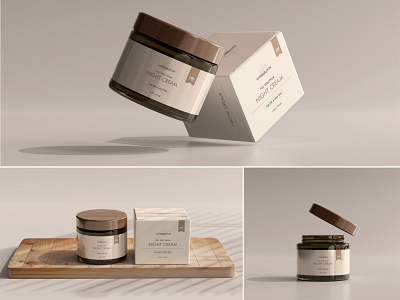This is a detailed digital collage featuring three distinct images of a night cream product. The largest image at the top displays a white-box package labeled "Night Cream" and a corresponding green canister with a brown lid, both hovering in mid-air at opposing angles, casting shadows against a white background. In the bottom left quadrant, the same cream-filled jar and its accompanying box are arranged on a wooden cutting board laid over a white surface. The bottom right image focuses on the canister alone, with the lid floating above it against an consistent off-white background similar to the rest. The detailed arrangement and varied perspectives highlight the packaging and presentation of the night cream, utilizing a palette of brown, white, tan, black, and gray tones to create a cohesive visual narrative.